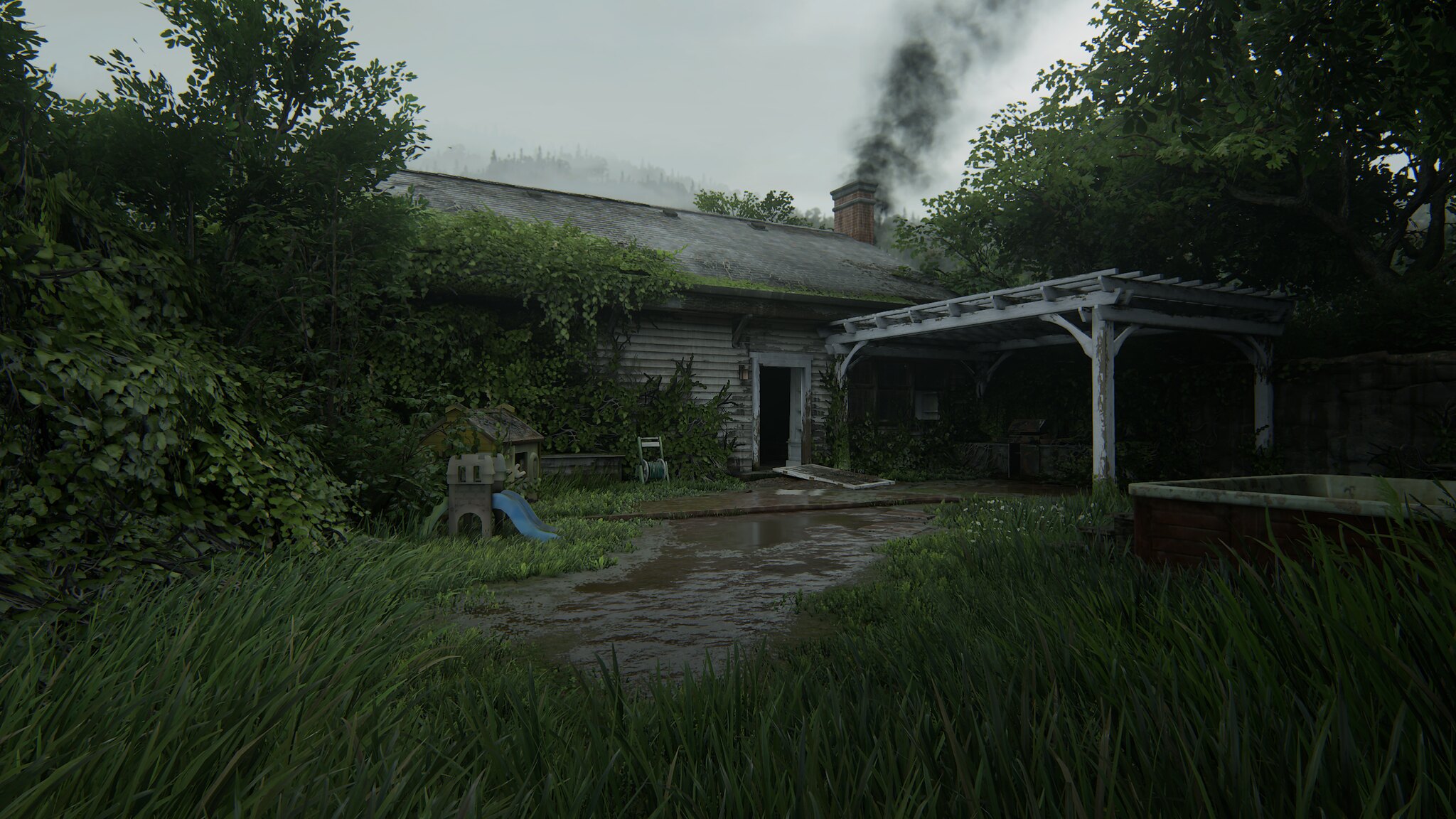In this eerily atmospheric photograph, we are presented with an exterior view of what appears to be an abandoned one-story house, likely either the front or rear. The home is clad in weathered white or light gray siding and is overshadowed by an overall gloomy ambiance of a possibly rainy day. The doorway prominently features a darkened frame, suggesting either a missing door or a pitch-black interior beyond.

A wooden canopy or trellis, visibly decrepit with peeling paint and signs of disrepair, extends from the house, evoking a sense of neglect. The roof, similarly aged and in need of maintenance, is topped by a brick chimney emitting black smoke, hinting at some occupancy within.

Nature appears to be reclaiming the structure, with ivy draping from the roof and creeping down the siding next to the door. Additionally, the house is enveloped by green moss, dense foliage, and tall grasses, giving it an overrun and almost enchanted appearance.

In the yard, we notice an old, dingy children's slide, adding an element of eerie nostalgia. The toy, somewhat resembling a small castle, is adorned with a distinctive blue spine and sits amidst a landscape dotted with trees and puddles from recent rain. The overall impression is one of dereliction and the quiet encroachment of nature on a once lively home.